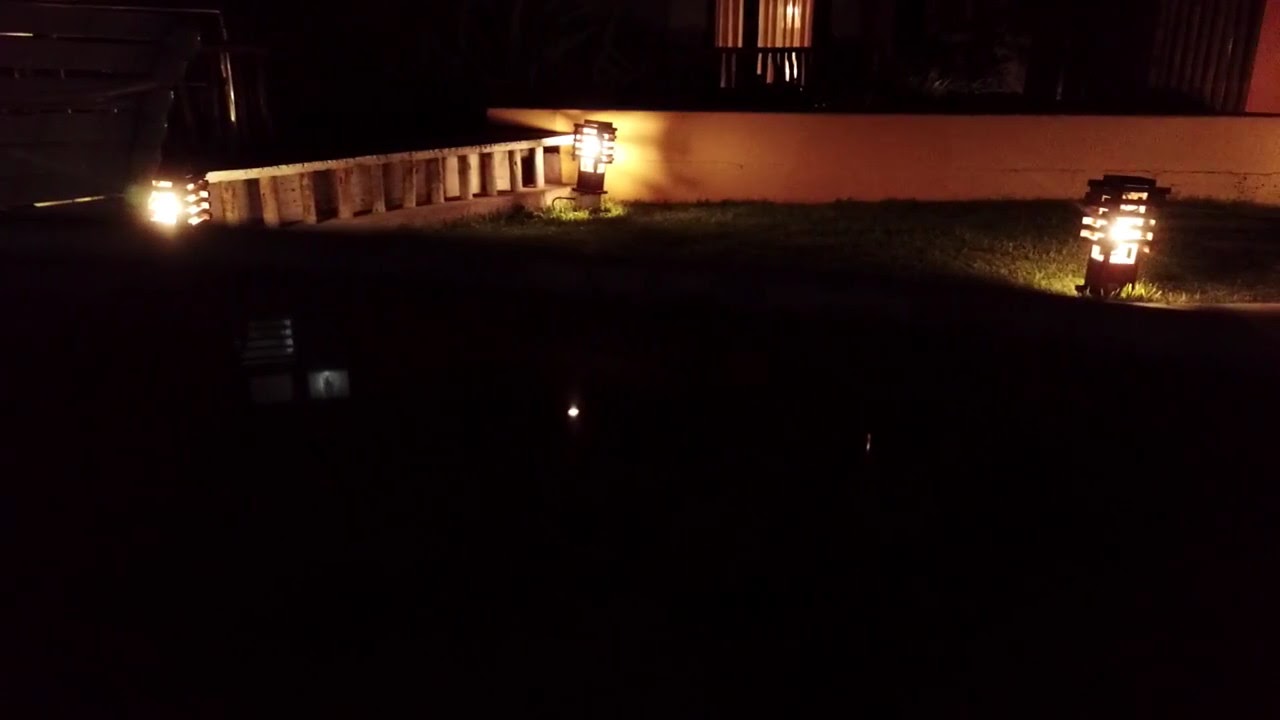This nighttime photograph captures a dimly lit yard scene, predominantly enveloped in darkness. A patch of short grass stretches across the foreground, which appears to be either a lawn or a park. Three small lantern-like yard lights planted in the grass stand out as focal points; two are lit, casting a muted glow, while one remains unlit. To the left and right of the image, there are additional light fixtures featuring dark lines, likely black light fixtures with lit bulbs. An off-white boundary wall or part of a house is visible in the distance, and to the left, another wall with possibly short bars, which might be steps or a patio, is partially discernible. The overall setting hints at a serene, albeit shadowed, yard space.